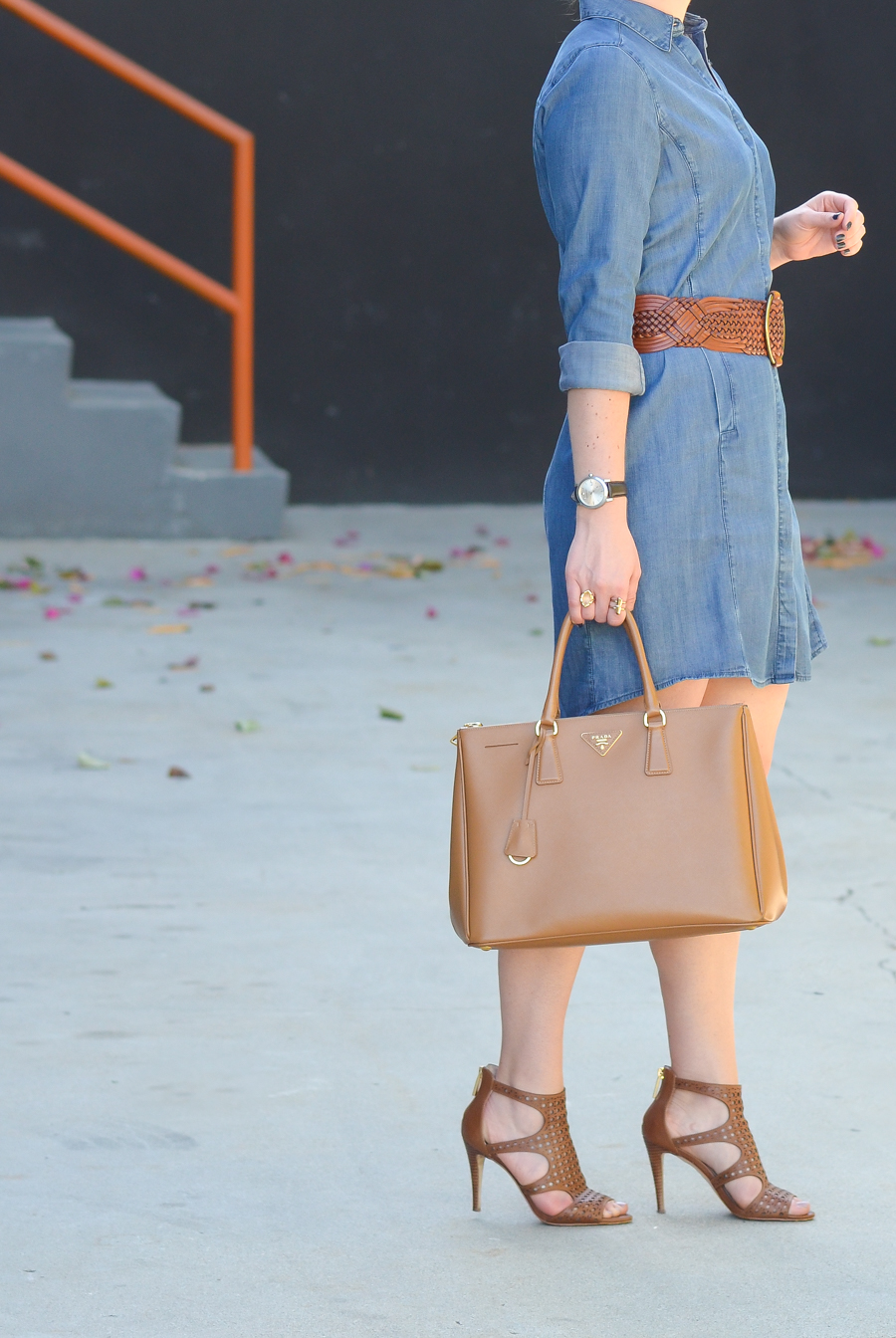This image captures a woman from the neck down, dressed in a blue denim shirt dress, featuring prominent stitching along the sides. She accessorizes with a brown leather belt that boasts a large, circular buckle. On her left wrist, she wears a watch with a brown band and a silver face. She is also adorned with a few rings and has her nails painted black. The woman holds a tan leather purse by its handles, which hangs down towards her legs. Her footwear consists of brown leather, open-toed heels with cutouts and a thin heel.

The setting features a gray concrete floor, scattered with debris that appears to be leaves in various shades of brown and orange. Behind her, a black wall serves as the backdrop. To the left of the frame, there are gray stairs complemented by an orange handrail. The scene is dominated by a color palette of blue, brown, gray, orange, and black.